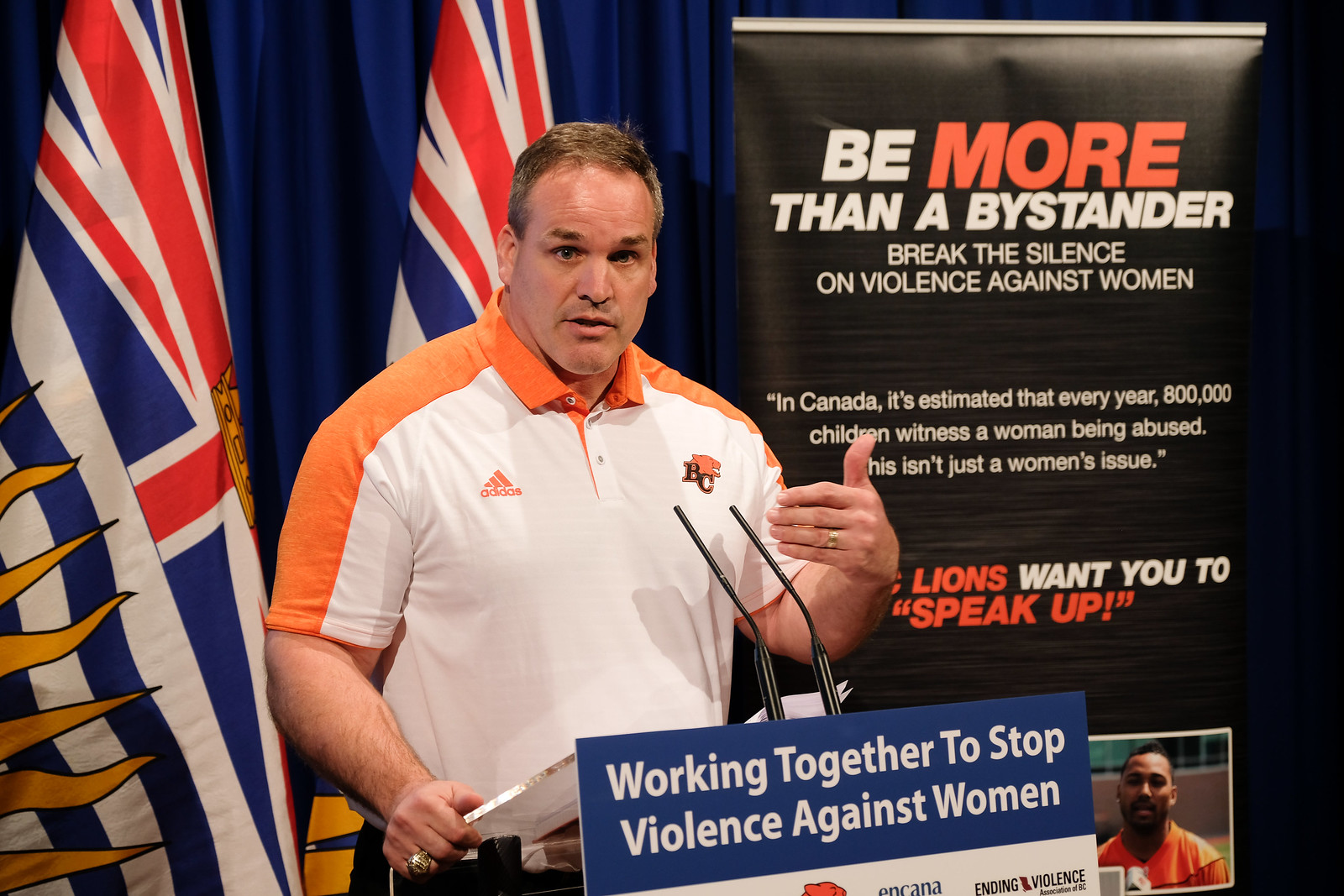In the image, a middle-aged, white-skinned gentleman with short brown hair stands behind a glass podium, addressing an audience. He wears a white polo shirt with orange shoulders and sleeves, adorned with the Adidas logo on the left and "BC" with an orange tiger logo on the right, suggesting he is a coach. His left hand is out in front of him, and his right hand holds some pages, with a silvery ring visible on his wedding finger. 

The podium features a placard with white text on a blue background that reads "Working together to stop violence against women." Behind him, there are a couple of Canadian flags against a blue curtain backdrop. Additionally, a prominent black roll-up poster stands beside him, displaying the message "BE MORE THAN A BYSTANDER" in large orange and white uppercase letters. Below that, it states "Break the silence on violence against women," with further details about domestic violence in Canada. The poster also highlights that the Lions encourage speaking up against violence. 

The overall scene suggests a campaign or initiative against domestic violence, championed by the speaker, who appears to be emphasizing the importance of standing up against such abuse.